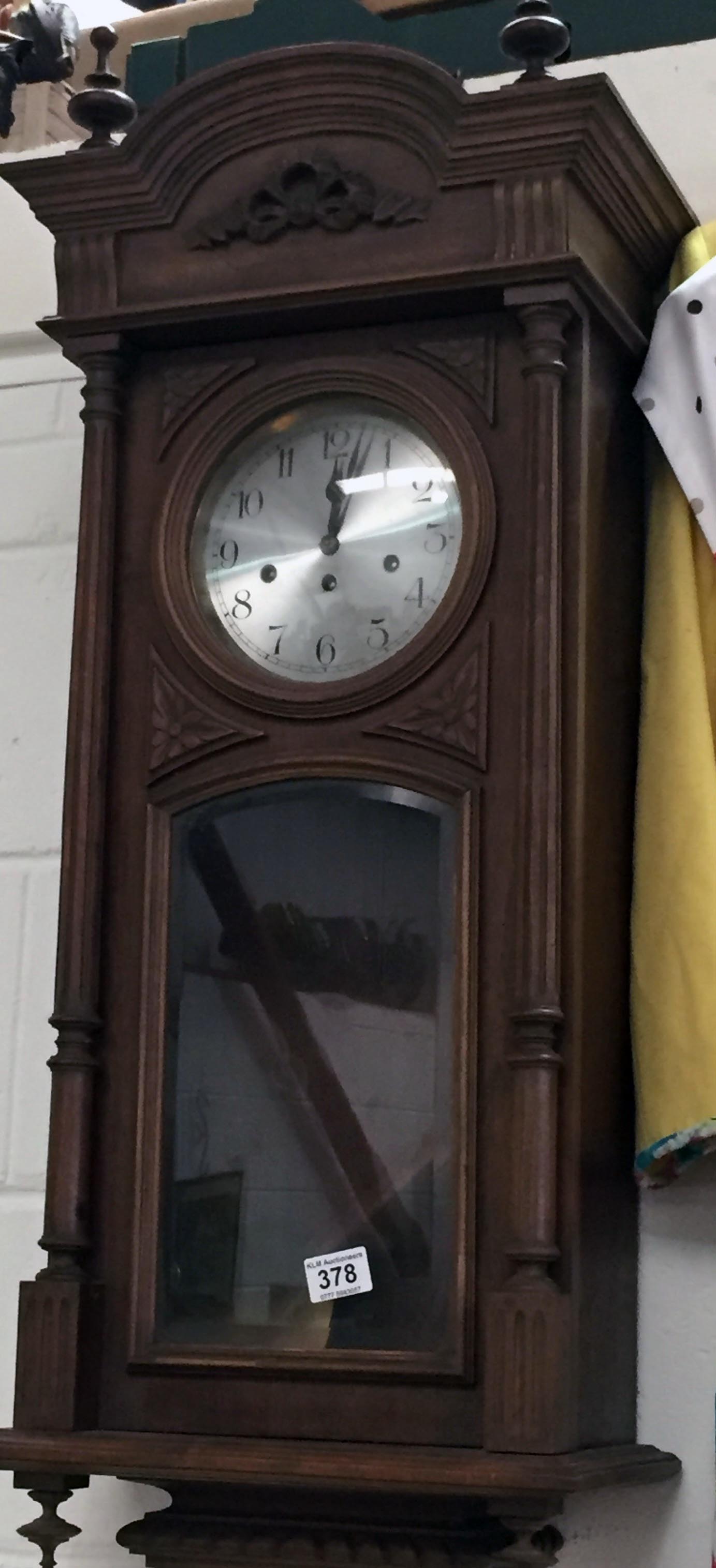The image features a background made up of white cinderblocks. At the top of the cinderblock wall, there's a light brown and green object, possibly a shelf holding various items. On the right side of the frame, a raincoat is hung up on the wall, displaying vibrant colors of yellow, green, and white. Additionally, a dark brown wooden clock with a round silver face is mounted on the wall. The clock includes an arch-shaped glass panel with vertical sides, through which a pendulum is visible. A rectangular sticker showing the numbers "378" is affixed to the front of the glass.